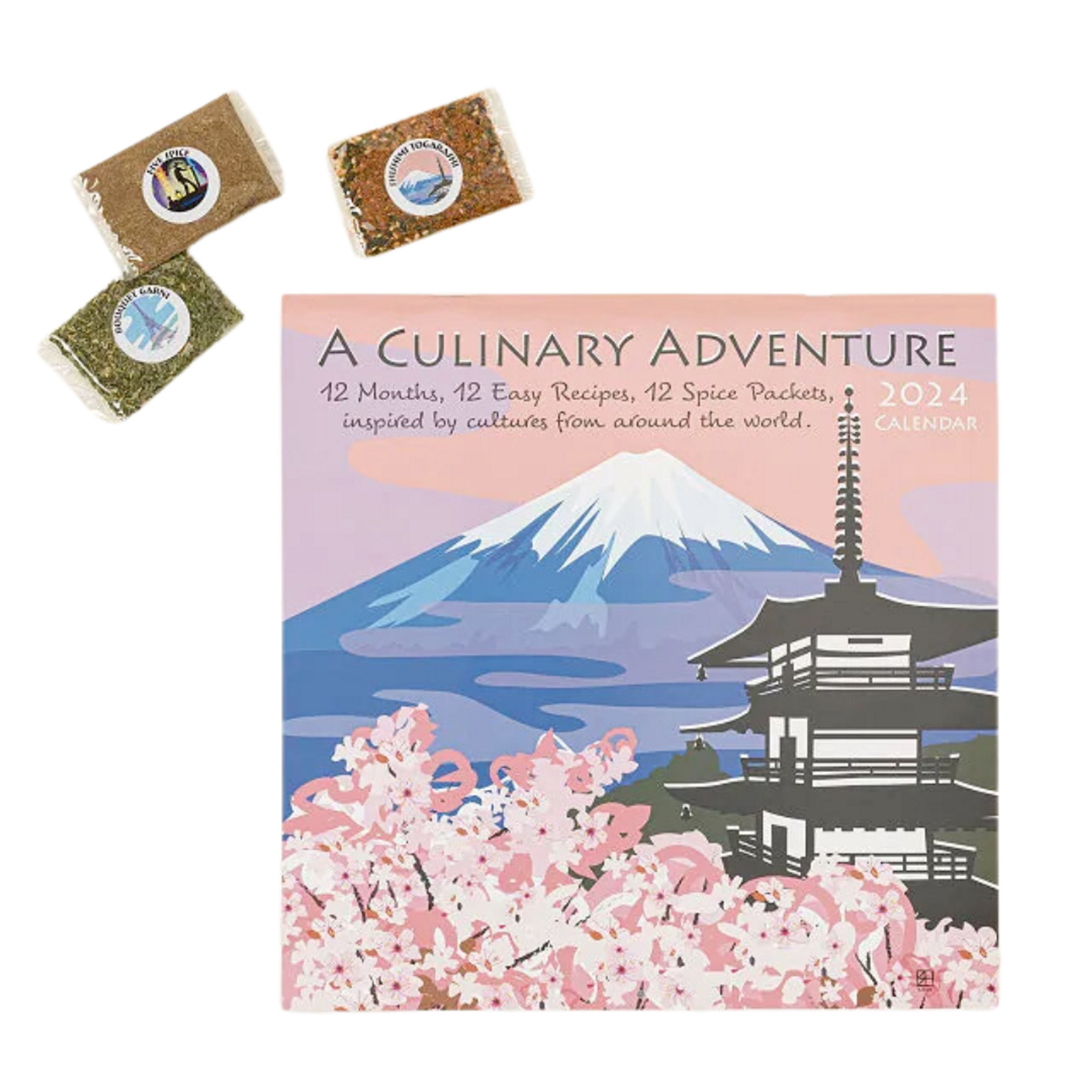This image features the cover of a "Culinary Adventure 2024 Calendar" prominently displayed on a pastel pink and purple background adorned with whimsical purple clouds. The poster, occupying the majority of the image's right side, is vibrant with a blue snow-capped mountain reminiscent of Mount Fuji, surrounded by ethereal purple clouds. In the forefront, a tree bursts with delicate cherry blossoms in shades of pink and brown, their fine branches stretching towards the sky. Nestled between the mountain and the cherry blossoms is a traditional pagoda-style building, rendered in dark gray and white, showcasing at least four levels with ornate balconies. The calendar boasts the text in muted gray font, stating, "A Culinary Adventure. 12 months, 12 easy recipes, 12 spice packets inspired by cultures from around the world. 2024 Calendar."

In the top left corner of the image, three small spice packets are displayed, each featuring a unique circular logo that alludes to different global cuisines. The spices include a green packet, a brown cinnamon-colored packet, and a packet with a mix of black and reddish spices peppered with lighter hues. The background palette features soft peach, lavender, and pastel shades, creating an inviting and adventurous culinary atmosphere.